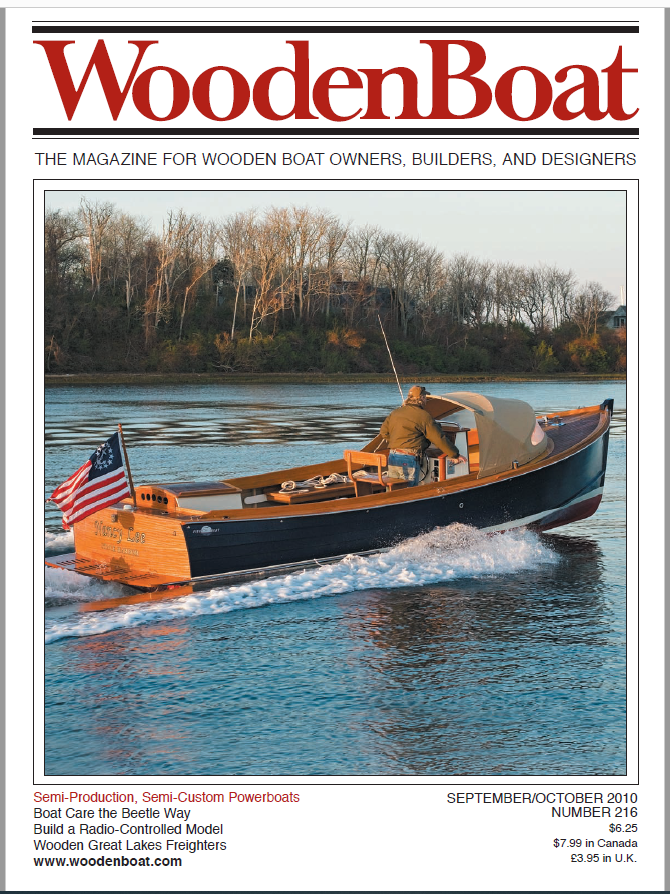The front cover of the September-October 2010 edition of "Wooden Boat" magazine (No. 216) prominently displays the title "WOODEN BOAT" in red capital letters, flanked by thick and thin black border lines. Below the title, in all caps, it announces: "THE MAGAZINE FOR WOODEN BOAT OWNERS, BUILDERS, AND DESIGNERS."

The main image captures a scenic moment of a wooden boat, blue in color and capable of seating eight to nine people along its benches. The boat, named with partially legible text reading "Missy", is skippered by a man in a green coat, brown hat, and jeans, standing and steering. The boat features a small canopy at the front, providing shelter from the elements, and an enigmatic flag with red and white stripes, a blue corner, and white stars in a circle—with an unidentified symbol at its center—fluttering at the stern. The tranquil backdrop reveals a landscape of trees and houses, enhancing the serenity of the scene.

In the lower section of the cover, the left side lists various articles in red and black text: "Semi-Production, Semi-Custom Powerboats," "Boat Care the Beetle Way," "Build a Radio-Controlled Model," "Wooden Great Lakes Freighters," and the magazine's URL www.woodenboat.com. On the right-hand side, the publication details are specified: "SEPTEMBER/OCTOBER 2010," "NUMBER 216," with pricing listed as "$6.25 USD, $7.99 CAD, £3.95 UK."